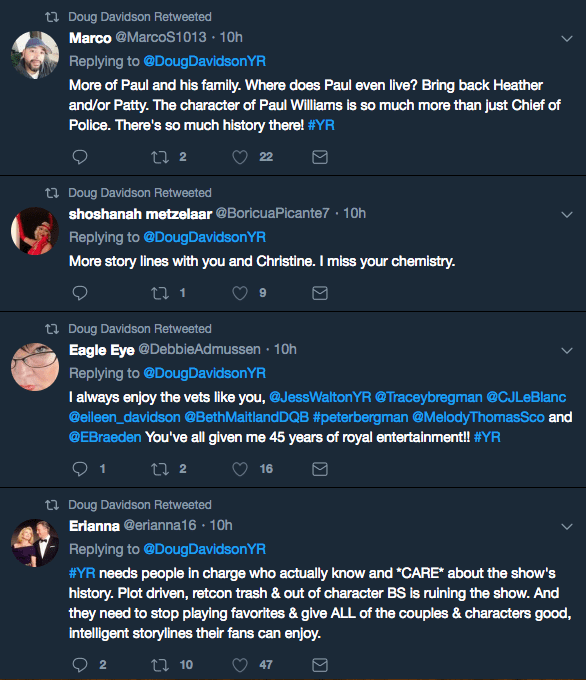This image displays a series of retweeted Twitter conversations involving actor Doug Davison, noted for his role as Paul Williams on "The Young and the Restless." The first tweet, retweeted by Davison from user Marco (@MarcoS1013), is a reply to Doug Davison YR from 10 hours ago. It reads, "More of Paul and his family, where did Paul even live? Bring back Heather and/or Patty. The character of Paul Williams is so much more than just Chief of Police. There's so much history there." This tweet has garnered 2 shares and 22 likes.

Below that, another retweeted tweet from Shoshanna Metzlar (@BoricuaPicante7) also replies to Doug Davison YR from 10 hours ago. It says, "More storylines of you and Christine. I miss your chemistry." This tweet has 1 share and 9 likes.

The final retweet in the image is from Eagle Eye (@DebbieEdmondson), again replying to Doug Davison YR from 10 hours ago. It states, "I always enjoyed vets like you, Jeff Walton YR, and Tracy Brinkman."

Each conversation highlights fan desires to see more of Davison's character and nostalgic appreciation for the veteran actors on the show.